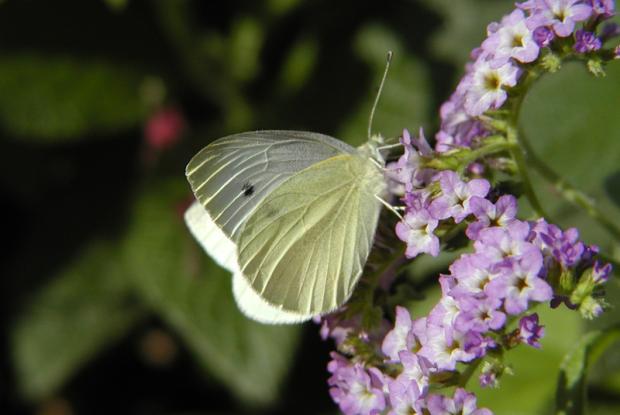This image captures a delicate butterfly or moth perched on a cluster of light purple, lavender flowers. One wing displays a creamy, pale green hue with a notable black dot, while the other wing appears more gray-green. You can observe the intricate shape of the antennas, adding to the insect's detail. The image is beautifully lit by the sun, casting subtle shadows on the insect's wings and creating a bright, sunlit effect. The flowers are abundant, each with white and yellow star-shaped centers, forming a cascading spray that loops around towards the top right of the frame and descends towards the center and bottom right. The background fades into a soft blur of green leaves and a distant, pinky-red dot, drawing focus to the butterfly and the flowers. This vibrant and detailed composition showcases the harmony of nature in a sunny setting.